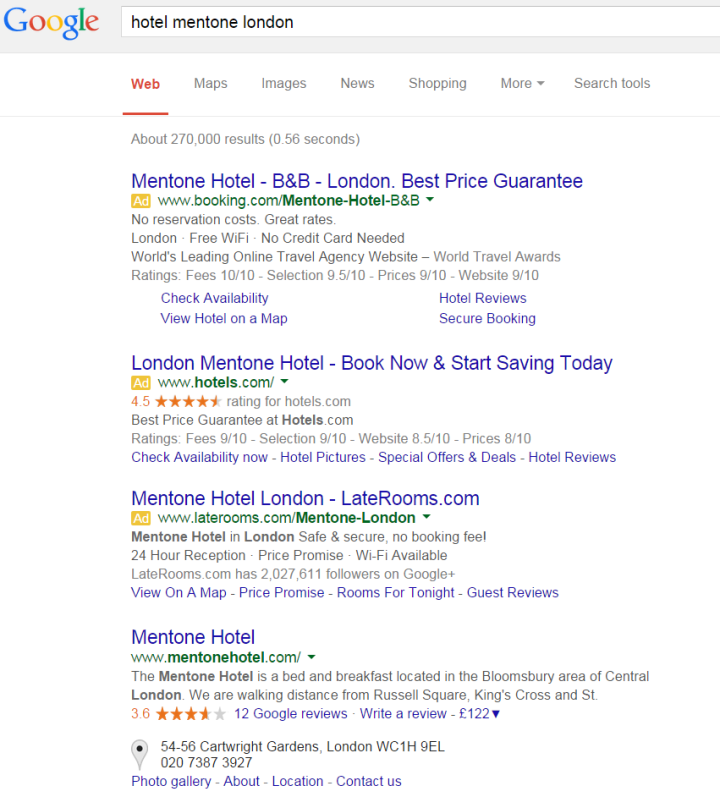A detailed Google search results page for "Hotel Mentone London" is displayed. The search query appears at the top within the search bar, and the screen features multiple navigational tabs including "web," "maps," "images," "news," "shopping," and "more," with "web" being highlighted in red, indicating the current active tab. Below, the results reveal approximately 270,000 entries, retrieved in just 0.56 seconds. The top search results include:

1. A link to the "Mentone Hotel, B&B London" featuring a best price guarantee.
2. A link titled "London Mentone Hotel" with options to book now and start saving.
3. A third link points to "Mentone Hotel London" on laterooms.com.
4. The final notable link lists the "Mentone Hotel" along with its address at 54-58 Cartwright Gardens, London WC1H and the contact number 020 7387 3827.